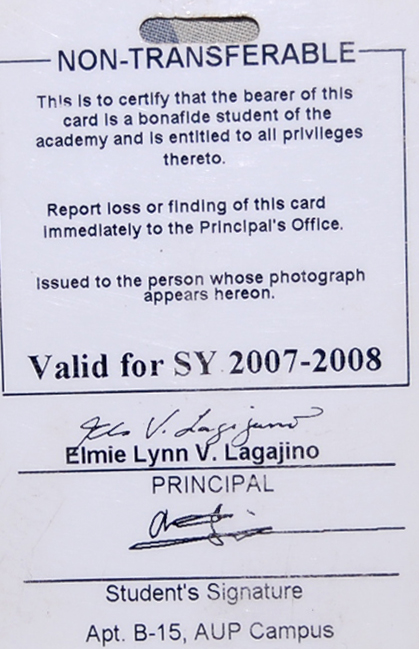The image features a white identification card with an oval hole punched out from the top. Centrally, there is a black square containing multiple lines of black text. It reads: "NON-TRANSFERABLE. This is to certify that the bearer of this card is a bona fide student of the academy and is entitled to all privileges thereto. Report loss or finding of this card immediately to the principal's office. Issued to the person whose photograph appears hereon. Valid for SY 2007-2008." Below the black square, there are designated areas for signatures. The first line displays the printed name of "Elmi Lynn V. Lagagino," with the label "Principal" and what appears to be the principal's signature above it. Below this, there is another line for the student's signature. At the bottom of the card, the text "APT B-15 AUP campus" is displayed, marking the student's residential address. The card is primarily gray in color aside from the clearly defined black text and the structure detailed above.